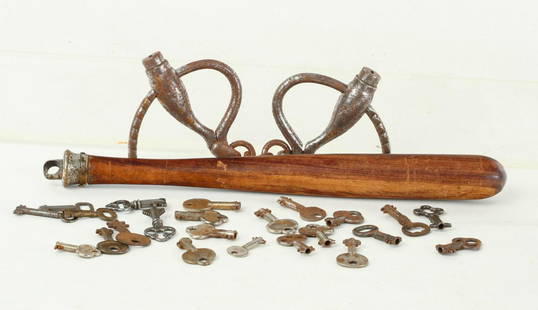The image is a color photograph set against a white background, without a border, signature, or date. Prominently featured in the center is a wooden baton, light brown with darker streaks at its end, and outfitted with a metal fastener near the handle. Behind the baton, there are two circular metal objects that resemble shackles or handcuffs, complete with lock mechanisms. In the foreground, scattered in front of the wooden baton, is an array of metal keys, varying in size, shape, and color—some are silver, gold, copper, with some keys featuring one or two holes of different sizes on their tops. This collection of objects, including the wooden baton and the possible shackles, suggests it could be vintage police equipment, perhaps used by peace officers in a prison or on the streets.